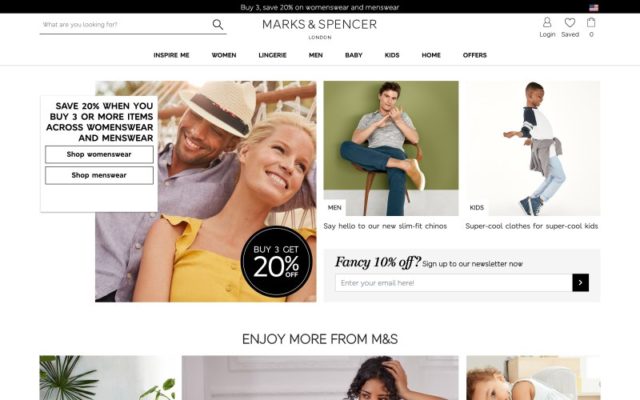Certainly! Here is a cleaned-up and detailed caption for the provided image:

---

The image showcases the landing page of an online clothing store, Marks & Spencer, against a predominantly white background. At the top of the page is a long, black rectangular bar displaying a promotion: "Buy One, Save 20%." To the right of this bar, an American flag indicates shopping from the United States portal of the website.

Below the promotional bar, the store's name "MARKS & SPENCER" is centrally positioned in bold capital letters. To its left is a search option labeled "What are you looking for?" accompanied by a magnifying glass icon. Moving to the right, there are options for login, saving favorite items, and a shopping cart.

Beneath this header, a menu bar offers various categories: Inspire Me, Women, Lingerie, Men, Baby, Kids, Home, and Office.

The central image features a promotional graphic with a man and a woman lounging on a hammock. The man, a young African-American in his early 30s, wears a tan fedora and a button-down shirt, smiling warmly with his arm around his companion. The woman, a similarly aged Caucasian with blond hair pulled back, wears a bright yellow shirt and also smiles. Text within this image reads: "Save 20% when you buy three or more items across women's wear and men's wear," accompanied by links to shop for women's wear and men's wear. The bottom corner of this image reiterates the offer: "Buy three, get 20% off."

To the right, another image promotes men's new slim-fit chinos. A young man, possibly in his late 20s, is seated on a wooden chair against a green background, wearing a button-down shirt, blue pants, and beige shoes, with his arms resting on the chair. Beside him stands a young African-American boy around 10 or 11 years old, dressed in light blue jeans, a gray sweater draped over his shoulders, a white shirt with blue sleeves, and blue sneakers. The caption for this section reads: "Kids: Super cool clothes for super cool kids."

Below these images is a call-to-action box encouraging visitors to sign up for the newsletter with an offer of "10% Off." It includes a field to enter an email address and a submit arrow button.

At the bottom, a caption states "Enjoy more from M&S," accompanied by three partially visible images: one hints at an artificial palm tree, the second shows part of a young woman with her hand in her hair, and the third depicts a glimpse of a girl's side profile and arm.